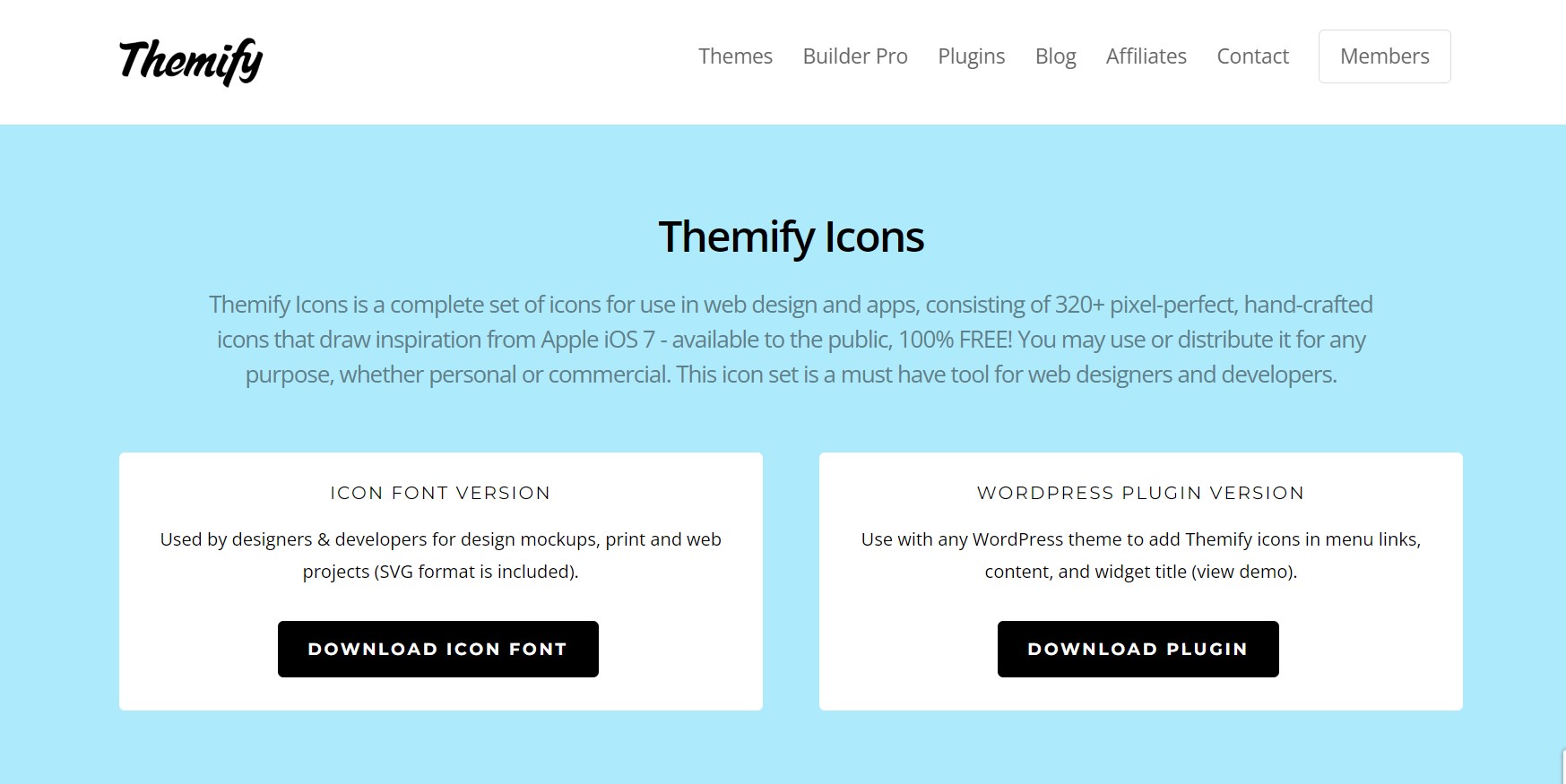**Detailed Caption for the Image:**

The image is sourced from the Themify website, showcasing its top navigation bar with clickable links leading to various sections: Themes, Builder Pro, Plugins, Blog, Affiliates, Contact, and Members. The backdrop features a light tealish-blue hue, providing a calming visual experience. Dominating the upper portion of the image is a blue rectangle box with the prominent title "Themify Icons." Beneath this in smaller font is a descriptive text revealing that Themify Icons is a comprehensive collection of over 320 meticulously designed icons inspired by Apple iOS 7. These icons are available for free use in both personal and commercial projects, making them an invaluable resource for web designers and developers. The lower portion of the image highlights two download options: "Download Icon Font" on the left and "Download Plugin" on the right, both in black buttons with white text.